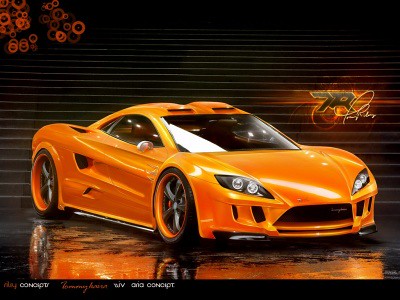This full-color, highly detailed image focuses on a stunning bright orange sports car with an ultra-modern aerodynamic design. The car's impressive features include doors that open upward, a sharply sloped windshield, and multiple spoilers adorning the top. The car's body and even its rims share the same striking orange color. Positioned on a reflective surface, the vibrant orange hue is mirrored beneath the car, enhancing its dramatic appearance. In a largely dark setting, the car stands out brilliantly against a backdrop that hints at a luxurious, perhaps futuristic environment—complete with intricate gold designs resembling gears in the upper left corner. Additional noteworthy elements include some text scattered across the image, with "7R" prominently displayed on the right side and a white signature nearby. The car, beautifully captured either in a photo or as a meticulously crafted computer-generated graphic, is showcased as if on a stage, suggesting a high-end marketing presentation. Small, unreadable print at the bottom and circles emanating from the upper left add to the sophisticated, high-tech ambiance of the scene.